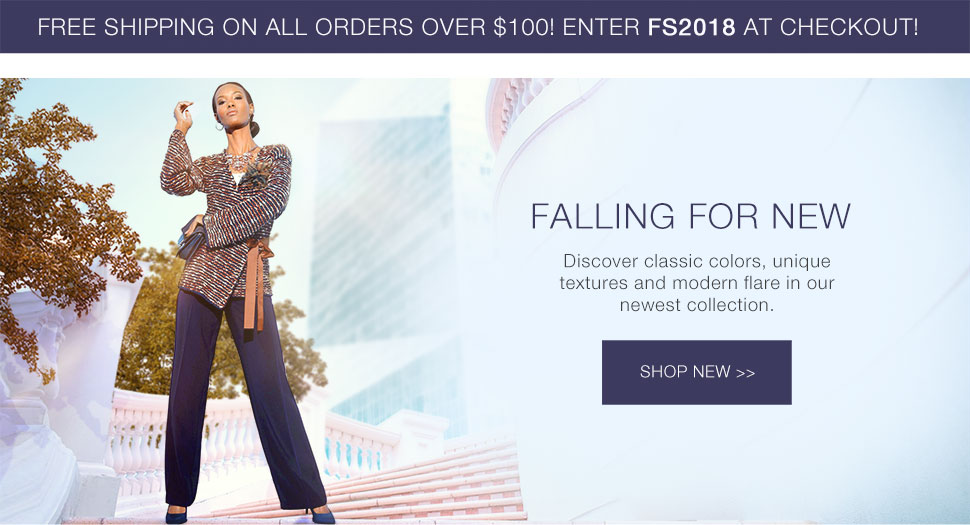In the image, the background transitions from a dark blue at the top to a lighter blue as it descends. At the top, a bold text reads, "Free Shipping on All Orders Over $100. Enter FS2018 at Checkout." Below this, the lighter blue backdrop showcases a woman standing elegantly. She is wearing a stylish multicolored top in shades of gray and brown, paired with blue pants and matching blue shoes. Surrounding her are trees, and the flooring beneath her has pink hues.

On the right side of the image, a promotional message reads, "Falling for New - Discover Classic Colors, Unique Textures, and Modern Flair in Our Newest Collection." Just below this, there is a dark blue button labeled "Shop New" with a double right arrow, inviting users to explore the new collection.

Overall, the image highlights a special offer on shipping and introduces a new collection with emphasis on classic and modern styles.